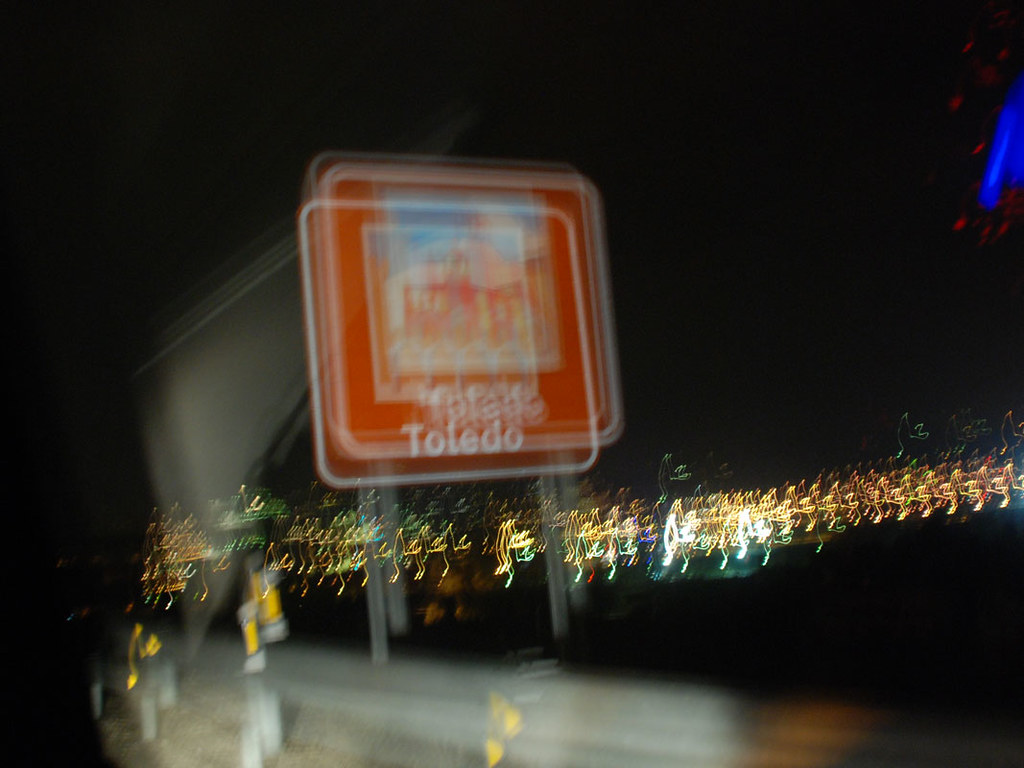The image captures a blurry scene taken at night, likely from inside a fast-moving car, showcasing a prominent road sign. The sign, which is rectangular with a white outer border and red interior, indicates the approach to Toledo, Spain. In the center of the sign is an indistinct picture of a monument, and the bottom part displays the word "Toledo" in white. Supported by two posts, the sign appears duplicated, creating a double-vision effect. Surrounding the sign are blurred city lights, forming streaks from the right to the bottom left corner, suggesting a vibrant cityscape. The road is flanked by a metal highway rail, colored grey with yellow sections. In the top right of the image, a blue beam of light with red flecks adds an element of mystery to the dark background.